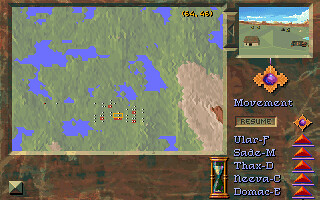The video game features a detailed map against a brown background. The landmasses on the map are depicted in vibrant green, while the bodies of water are a striking blue. An island, distinguishable by its lighter brown color, protrudes into the water. On this island, there is a brown square, and scattered across the map are small red and yellow characters. 

To the side of the main map, there is an illustration showing a scene with houses, roads, and cars. Above this scene, the word "Movement" is prominently displayed in white lettering. Additionally, the names Euler, Sade M., Thanks D., Neva, and Donik are also listed, providing special acknowledgments or credits.